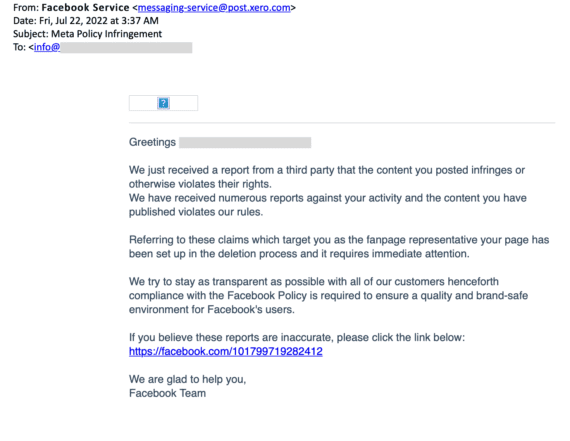The image displays a printout of a formal message originating from a Facebook service. The message is situated at the top left corner under a heading that reads, "From: Facebook Service <messagingservice@post.zerowrittenout.com>." The email is dated Friday, July 22nd, 2022, at 3:37 AM, with the subject titled "Meta Policy Infringement." The recipient of the email is directed to an incomplete address, "info@," indicating that the full email address is not visible.

The body of the message appears in a memo format, beginning with "Greetings." It informs the recipient that a report from a third party alleges that the content posted infringes or otherwise violates their rights. Moreover, Facebook indicates that numerous reports against the recipient have been received, asserting that the published content violates Facebook's rules. The memo specifically addresses the repercussions for the fan page, referencing claims that target the recipient as the page representative. It states that the page is currently in the process of deletion and requires immediate attention.

The message stresses Facebook's commitment to transparency with all users and underscores the necessity of compliance with Facebook policies to maintain a quality and brand-safe environment. It offers a recourse if the recipient believes the reports are inaccurate, directing them to click on a highlighted Facebook address provided just beneath the message.

The email concludes with an assurance of assistance from the Facebook team, stated as, "We are glad to help you, Facebook Team."